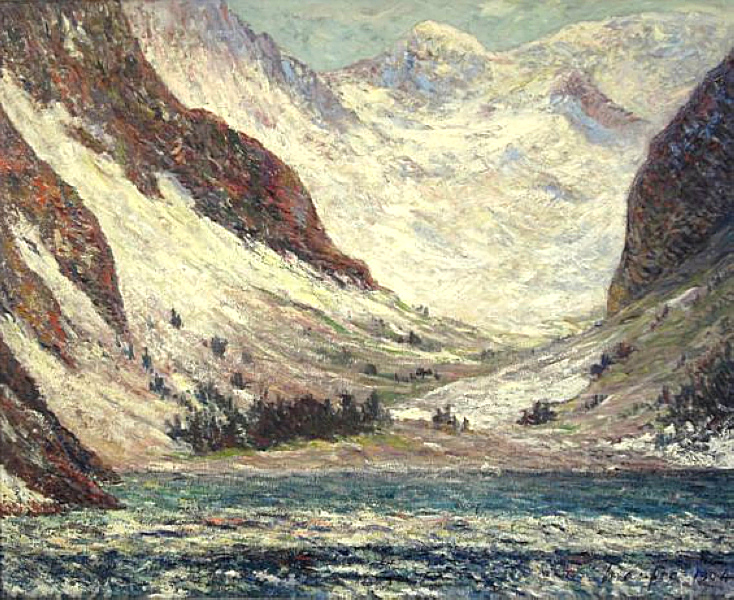This artwork depicts a breathtaking outdoor scene of a snow-covered valley flanked by imposing mountain ranges. In the foreground, a serene body of blue water, possibly a lake or river, occupies the bottom portion of the image. The water, with its teal and white frothy bits, meets a bank with scattered rocks, dirt, and clusters of vegetation, including some dark evergreen trees and light green grass. 

Above this, the valley stretches out with snow-dappled trees, and the scene is framed on either side by mountain slopes—the left slope tinged with a reddish-brown hue and the right partially hidden yet similarly snowy. Dominating the background is an immense snow-laden peak, its white expanses contrasting against a turquoise sky. The clear blue sky and snow seamlessly blend at the image's summit, enhancing the majestic beauty of this mountainous landscape. This piece, likely an oil painting, captures a vivid and tranquil natural environment with remarkable precision and artistry.